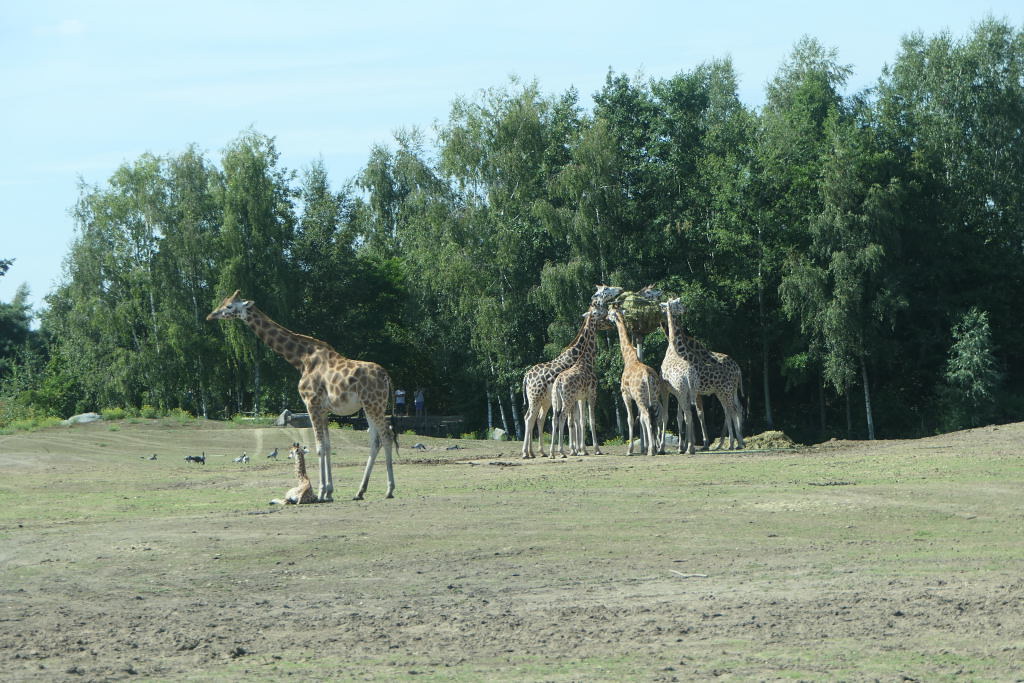This image captures a vast, slightly uneven field with patches of sandy dirt and low-cut grass, bathed in the light of a clear blue sky. Prominently featured in the center foreground is a large adult giraffe gazing off to the left, with a small baby giraffe lying at its feet. In the background, four giraffes are clustered together, forming a circle as if engaged in conversation. These giraffes, with their long necks and brown-and-white spotted coats, stand near or in front of a cluster of trees, adding to the natural ambiance. The distant left of the photo shows smaller animals resting on the ground, enhancing the scene’s sense of wildlife harmony. The overall setting appears to be the giraffes' natural habitat, offering a serene and picturesque glimpse of their lives in the wild.